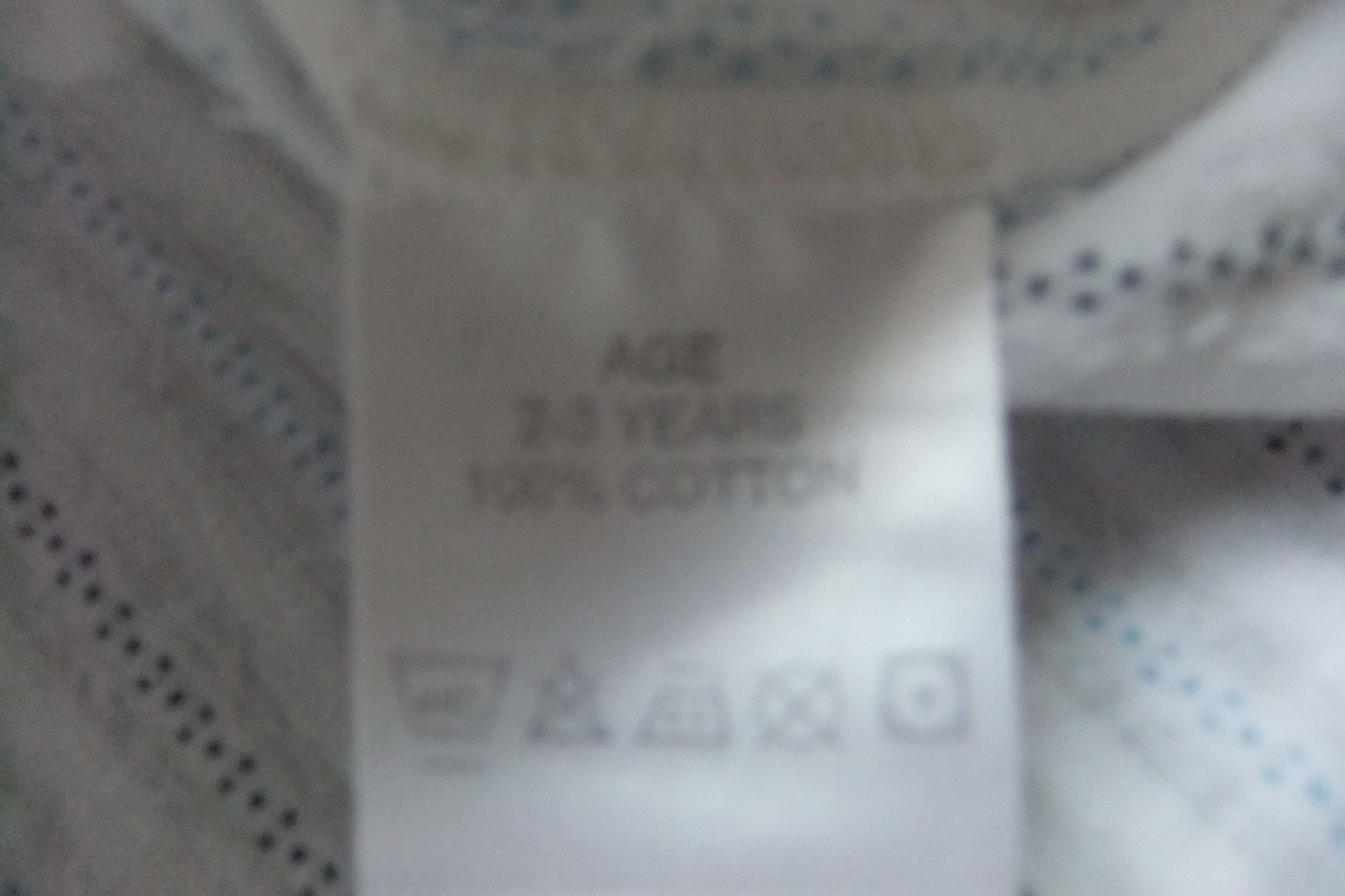A close-up view captures the manufacturer's tag on a toddler's garment, slightly shrouded in dim lighting, resulting in a somewhat blurry image. The white, satiny fabric tag is partially obscured by shadows, showing important details such as the recommended age "2-3 years" and the composition "100% cotton." Below this information are various care symbols indicating specific instructions on how to handle the fabric. The shirt itself appears to be exceptionally soft, featuring a horizontal gray and white striped pattern interspersed with small blue and green dots within some of the white stripes. The tag seems to be sewn into the collar of the shirt, subtly enhancing the garment's overall design.